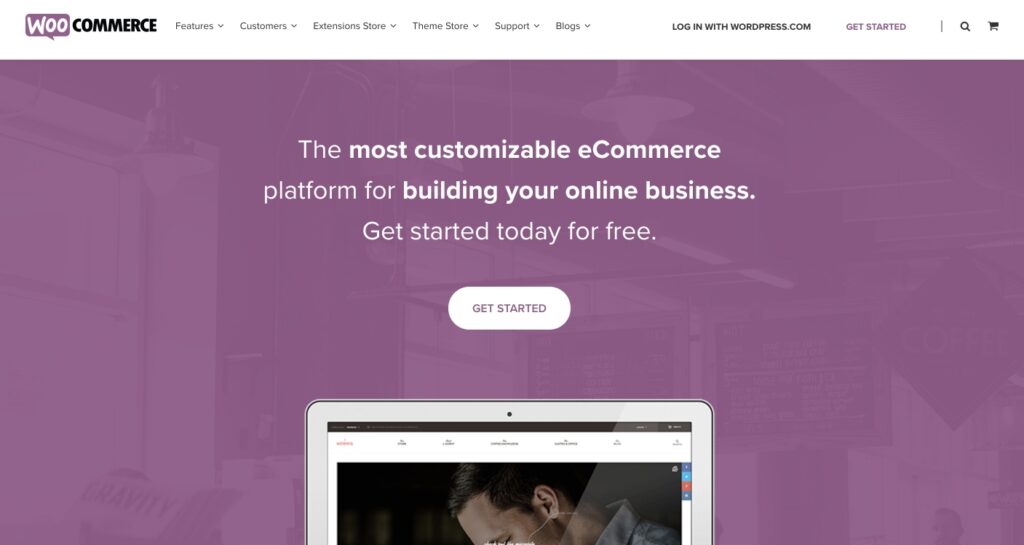This is a detailed description of a website's homepage, accessible via smart devices or computers.

The image features a horizontally oriented screenshot of the WooCommerce website. At the top, the background is a clean white, typical of a computer screen. Below this, the background transitions into a mauve color. The WooCommerce branding is prominently displayed: "Woo" is written in white letters set against a purple background, while "Commerce" is in black.

Just beneath the logo, there are navigation options, which include "Features," "Customers," "Extension Store," "Theme Store," "Support," and "Blogs." To the right of these options, "login with WordPress.com" is boldly labeled in black text. Adjacent to this is a mauve-colored button labeled "Get Started," followed by a vertical line, a search bar, and a shopping cart icon.

Further down, the background shifts to a purple-themed image featuring faint lights and building windows, not meant to be the focal point but adding some texture. Overlaid on this background, in white text, is the tagline: "The most customizable eCommerce platform for building your online business. Get started today for free." This call to action is accompanied by a rounded "Get Started" button.

At the bottom of the image, there is a depiction of a white device, likely an iPad, displaying a cropped image of a person, focusing on the top half.